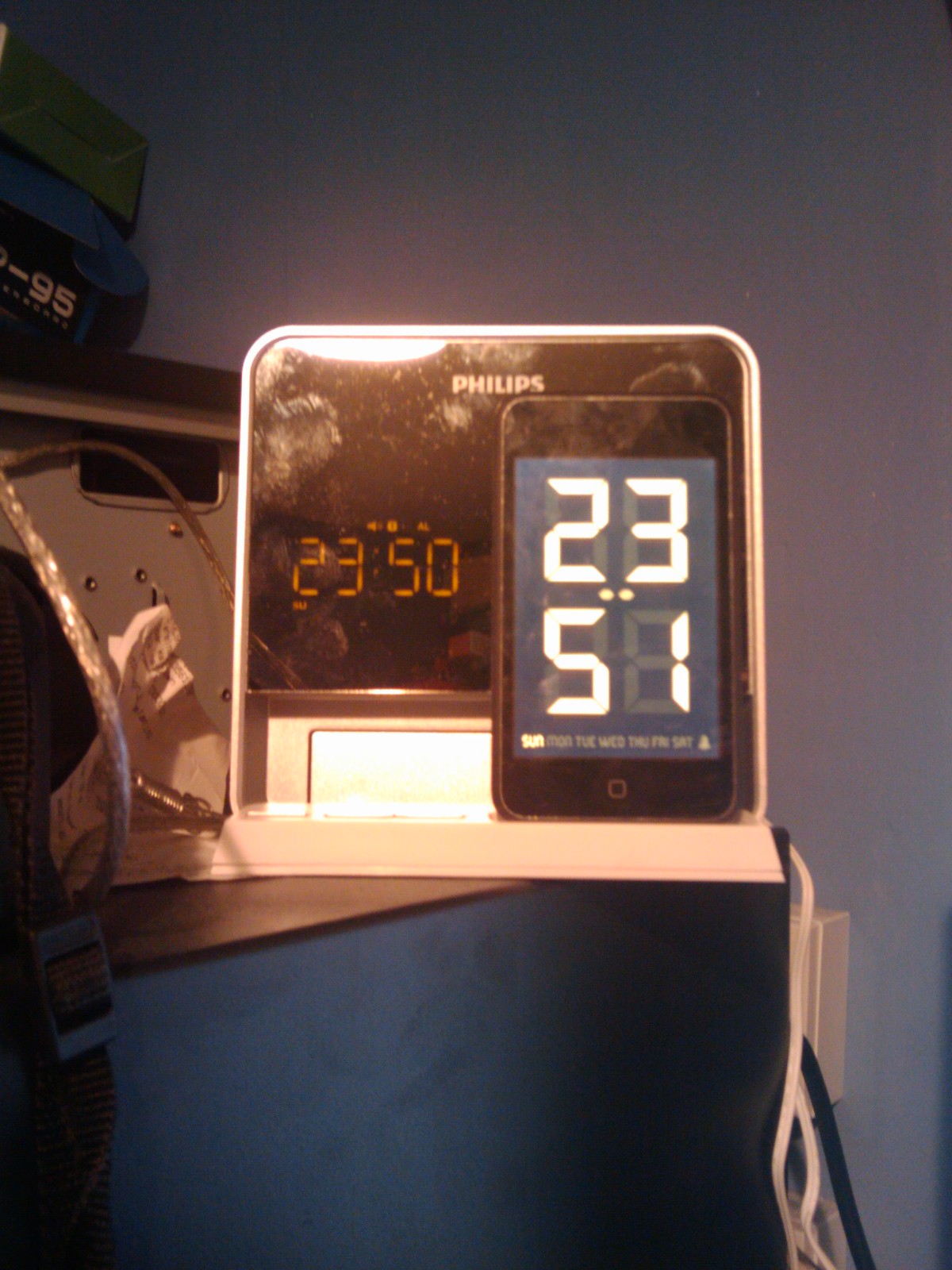The image displays a scene with a Philips digital clock and a smartphone showing the time. On the left, a Philips digital clock with a black screen prominently displays the time 23:50 in red numbers. The clock is positioned on a light bluish base. To the right, a smartphone, potentially a model with a single home button located at the bottom center, shows the time 23:51 in large white numbers along with "Sunday." This phone appears to be sitting on the same light bluish base as the clock. White cords can be seen trailing from the base toward a white outlet on the bottom right side of the image. The backdrop is a grayish color, reflecting some light, perhaps from a flash, clearly illuminating the Philips screen. On the left, there might be remnants of a book bag or a small purse, adding a subtle element of intrigue to the background.